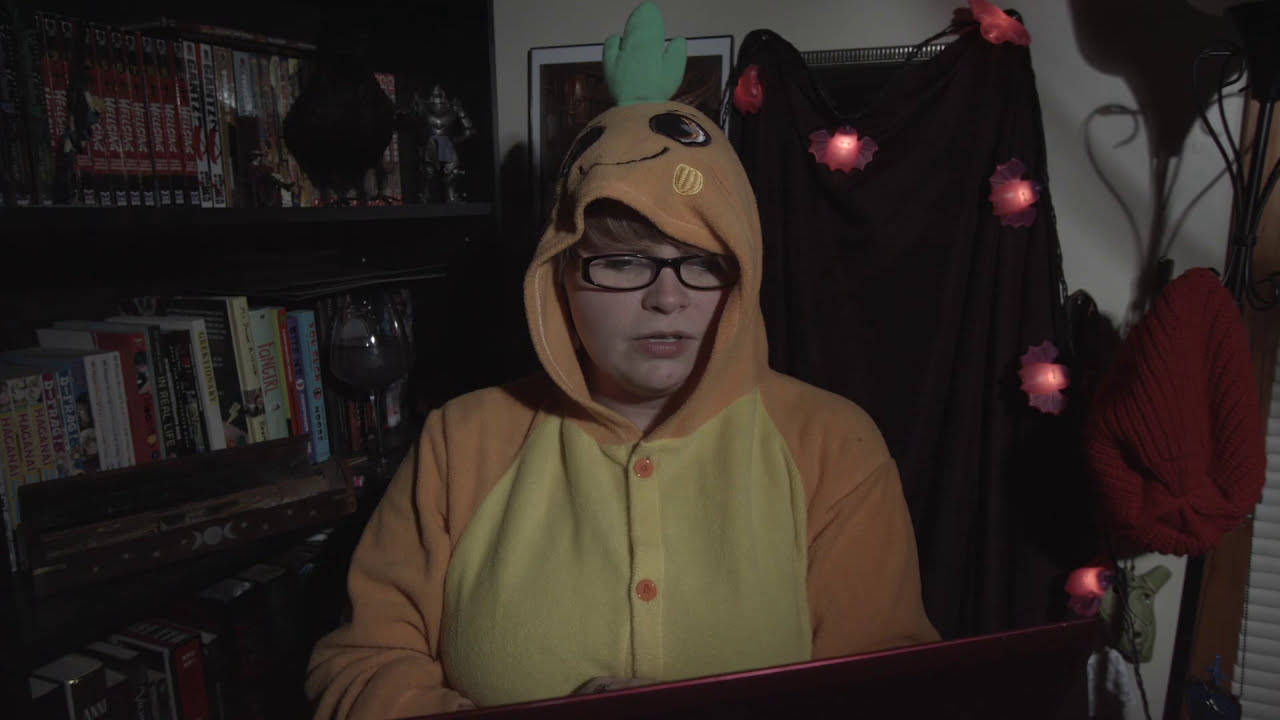In this dimly lit, indoor setting—possibly a bedroom or a recording studio—a person dressed in a vibrant costume takes center stage. The costume is a whimsical onesie, predominantly yellow with orange sleeves, featuring a hood that showcases eyes, a smiling mouth, and a tuft resembling a carrot stem or possibly a rooster crest. They wear black-framed glasses and hold a rectangular, partially red object in one hand. Surrounding the individual, the background reveals warm, homey details: a bookshelf on the left lined with rows of books, including a notable series with uniform spines and an ornamented figure of a medieval knight. Behind them, a black curtain decorated with illuminated, red, string lights—shaped like bats—adds a festive, cozy touch, hinting that this scene could be part of a vlog or podcast recording. The walls also feature hanging pictures, completing this charming and detailed visual tableau.